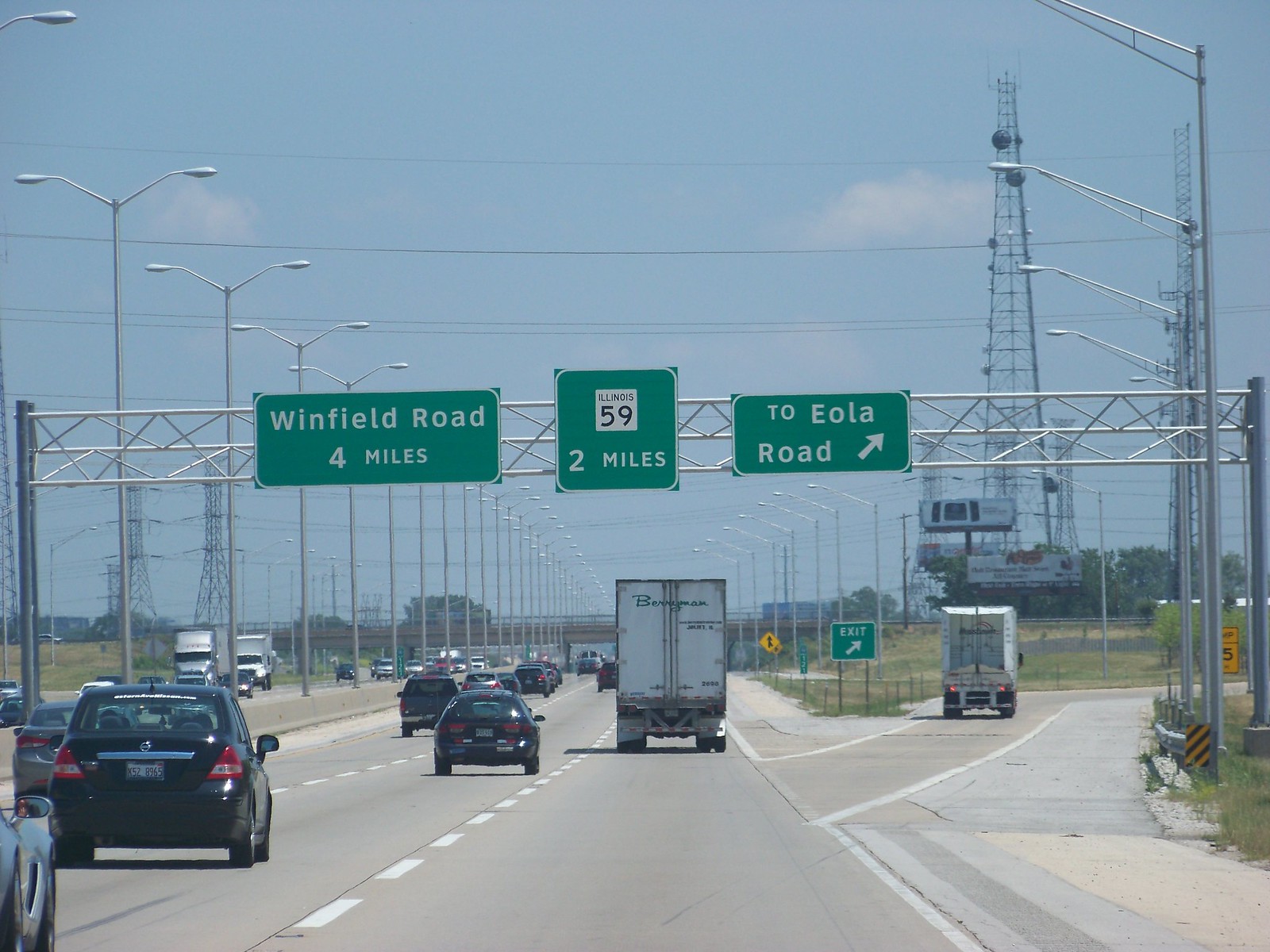This image captures a daytime scene on a multi-lane highway, likely taken from a dashboard camera inside a vehicle. The highway is divided by a median, with three lanes heading in each direction, and is bustling with traffic, including a noticeable big white truck and numerous other cars. An exit on the right shows a large truck taking the ramp. Overhead, the sky is a clear blue with some scattered clouds.

Prominent in the scene are multiple green street signs mounted on a steel girder beam. One rectangular sign directs drivers to Winfield Road in four miles. Another square sign indicates Illinois 59 is two miles ahead. The rightmost sign points towards an imminent exit to Eola Road with a white arrow. A detail worth noting is the numerous close-spaced streetlights and a signal or cell tower visible in the background. Additionally, there are power lines running across the top of the image and some grass seen along the right side of the road. The colors present in the image include various shades of blue, green, white, gray, silver, yellow, and black.